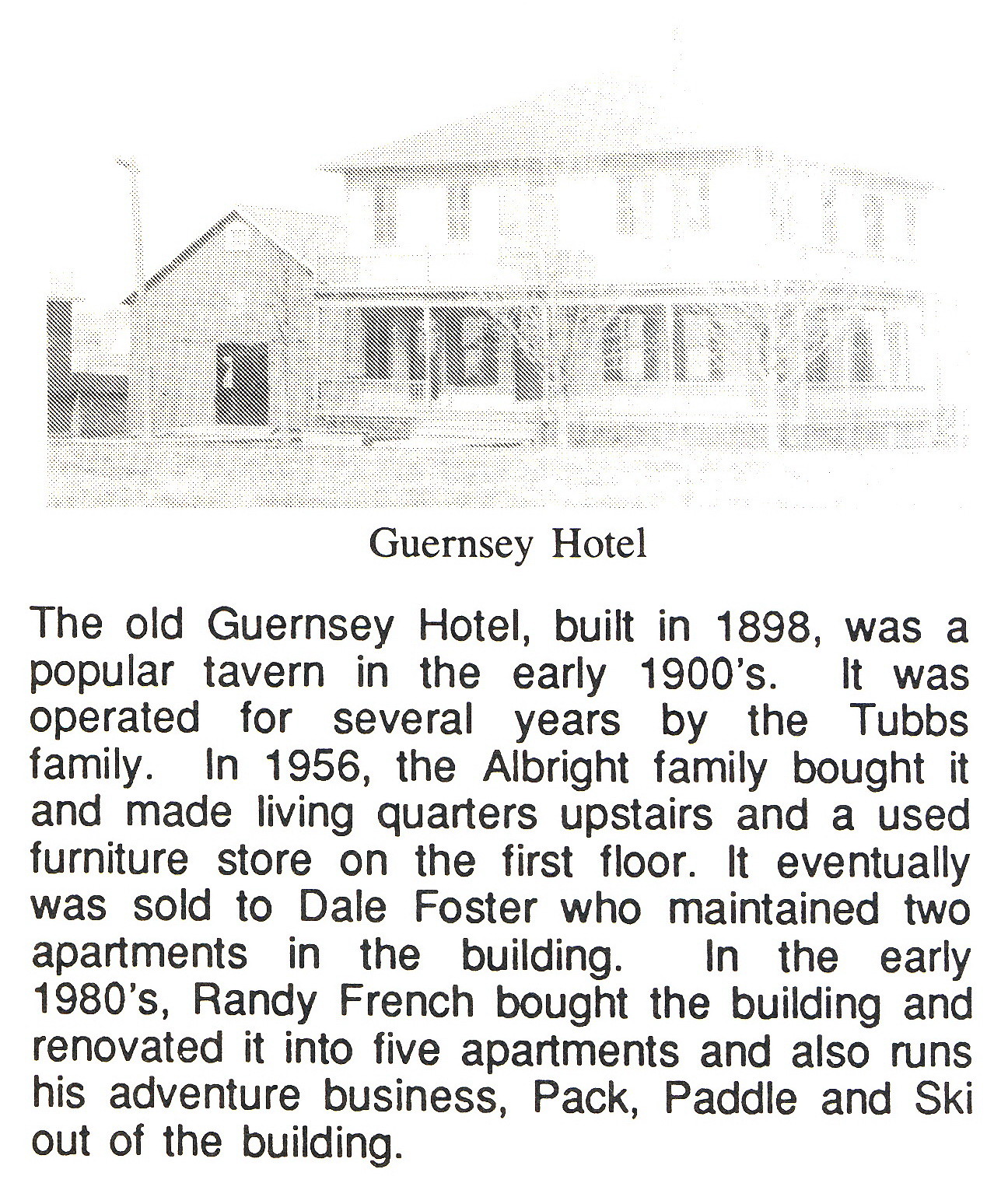The image is a rectangular, black-and-white, pixelated scan of a vintage advertisement for the Guernsey Hotel, blending into a plain white background. It features a dot-matrix styled, faded photograph of a two-story, ranch-style building with a sloped roof and a small, triangular-roofed shed to the left. Sparse trees are scattered in front of the hotel, adding to its old-timey charm. Below the photograph, in black print, the caption "Guernsey Hotel" is prominently displayed, followed by a detailed historical paragraph. The paragraph reads: "The old Guernsey Hotel, built in 1898, was a popular tavern in the early 1900s. It was operated for several years by the Tubbs family. In 1956, the Albright family bought it and made living quarters upstairs and a used furniture store on the first floor. It eventually was sold to Dale Foster, who maintained two apartments in the building. In the early 1980s, Randy French bought the building, renovated it into five apartments, and also runs his adventure business, Pack Paddle and Ski, out of the building." This comprehensive description encapsulates the rich history and various transformations of the Guernsey Hotel over the decades.